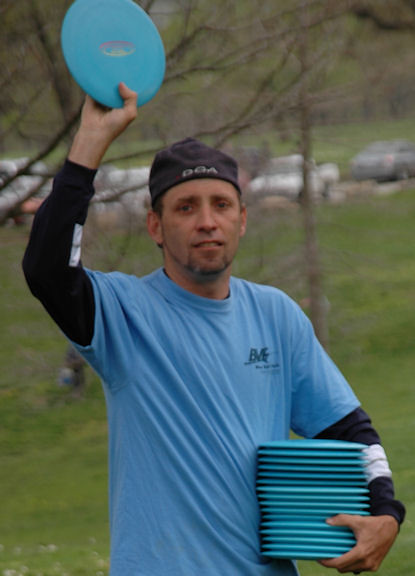This image captures a Caucasian man standing in a park-like setting, with green grass, leafless trees, and a parking lot filled with cars in the background. He is wearing a black beanie with the white initials "DGA" on it, a long-sleeve black shirt adorned with white squares on the arms, and a blue short-sleeve t-shirt with an emblem containing the letters "BVE" and some unreadable text over the left breast. His closely shaved hair and beard frame blue eyes that are looking directly at the camera. With his mouth slightly open, he holds up a light blue frisbee featuring a yellow and red logo above his head in his right hand. In his left arm, he clutches a stack of approximately 15-20 identical frisbees.